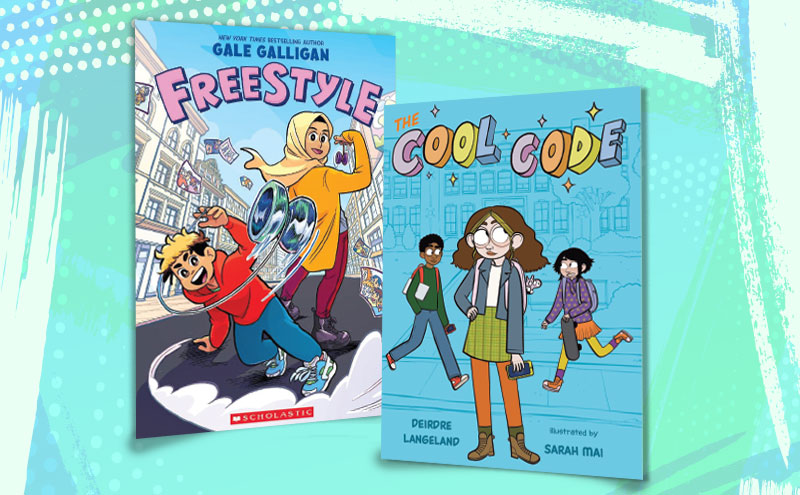The image shows two colorful comic book covers against a green background with white dots and paint-like marks. The left book is titled "Freestyle" by Gale Galligan, prominently displayed in pink lettering above the boy and girl on the cover. The boy has yellow hair, a red sweatshirt, blue jeans, and blue sneakers; he is throwing a yo-yo. Next to him stands a woman wearing a yellow hijab, a yellow sweater, a blue shirt, red pants, and black boots, also throwing a yo-yo. The Scholastic logo is visible in red with a white emblem. The right book is titled "The Cool Code," showcasing three kids. The central character is a girl with a jacket and backpack, holding a wallet, and appears to be rolling her eyes with a hand on her hip. To her left, a boy is dressed in a green shirt and blue pants, and to her right, a girl in a purple shirt and orange skirt holds a skateboard. Below the characters, it says, "Dear Dre Langeland" and "Illustrated by Sarah May" in smaller print. These vibrant and engaging covers highlight the playful and dynamic essence of the comics.